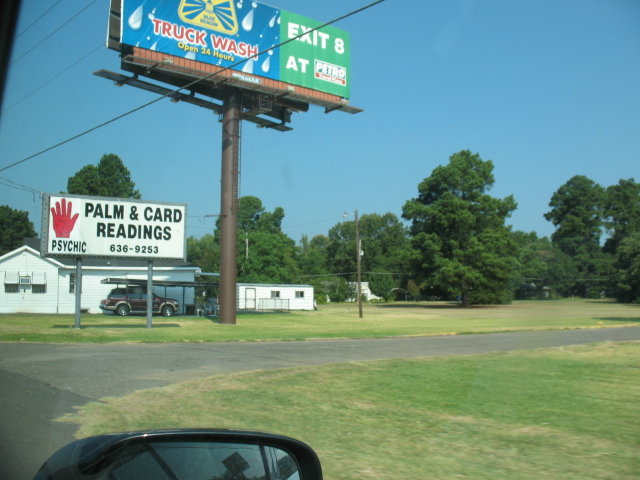Captured from the front passenger seat of a car, this photograph showcases a vibrant roadside scene under a clear blue sky. In the foreground, the car's black side-view mirror reflects the closed window, emphasizing the vantage point from within the vehicle. The image reveals an asphalt road cutting through a field of green grass. On the far side of the field stands a white building with gray wood paneling, beside which a red car with white trim is parked underneath a canopy, along with a white-paneled trailer to its right. Prominently featured are two billboards: the first, a small sign closer to the house, displays a red hand symbol and advertises "Palm and Card Readings," with the contact number 636-9253 and the word "Psychic" below. The second, a much larger billboard on a towering gray metal pole, announces "Truck Wash, Open 24 Hours" with "Exit 8" indicated, set against a blue backdrop adorned with water droplets. The distant background is lined with well-developed trees, completing this detailed and lively snapshot of a roadside vista.